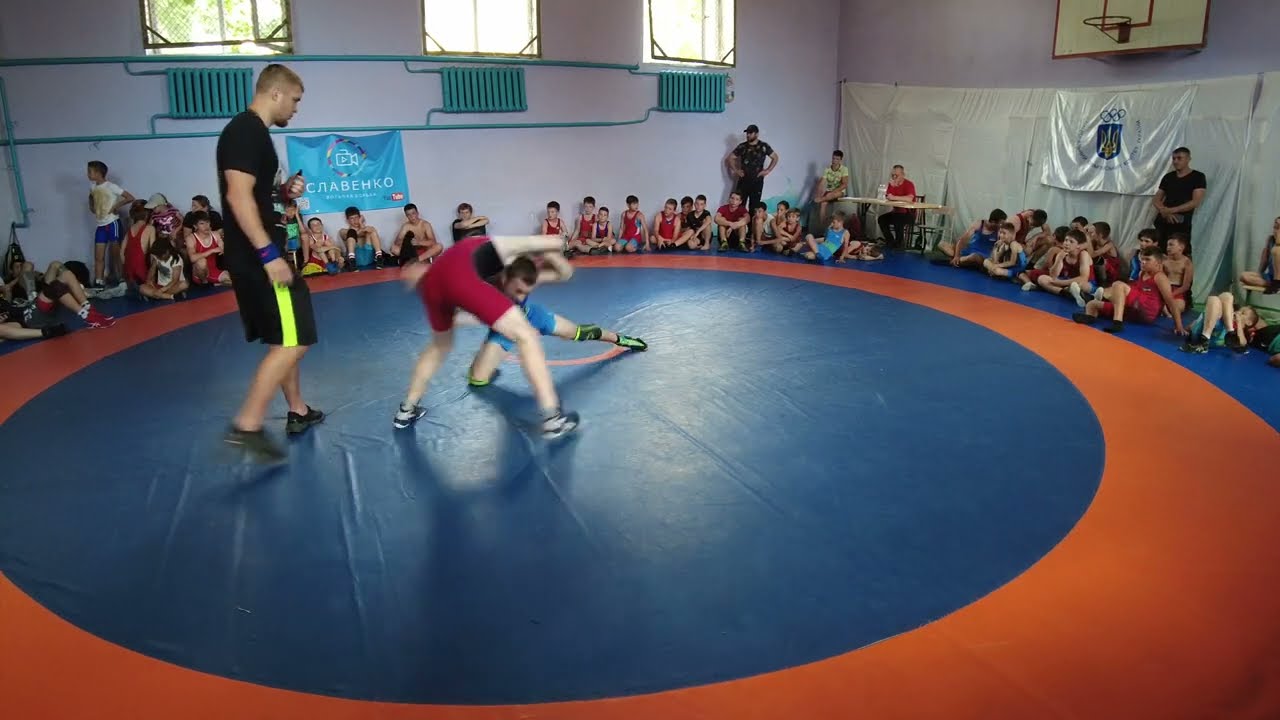The image captures an intense moment of a wrestling match in a gymnasium. At the center of a large blue wrestling mat with an orange outer circle, two boys are grappling—one in a red and black unitard, the other in blue and black. Overseeing the match is a referee, identifiable by his black shirt with a yellow stripe down his black shorts, black sneakers, and a blue wristband. He appears to be holding either a phone or a timer. The gym setting is clearly marked by white walls, a basketball hoop on one side, and blue radiators under windows. A banner with what looks like white Russian writing hangs on the far side. Surrounding the mat are spectators, including several children sitting and watching the match intently, with adults—possibly coaches or supervisors—standing nearby. On the right, a small table is occupied by two more adults, likely serving as judges for the match. The scene is indicative of a well-organized wrestling meet, with participants and observers alike fully engaged in the event.